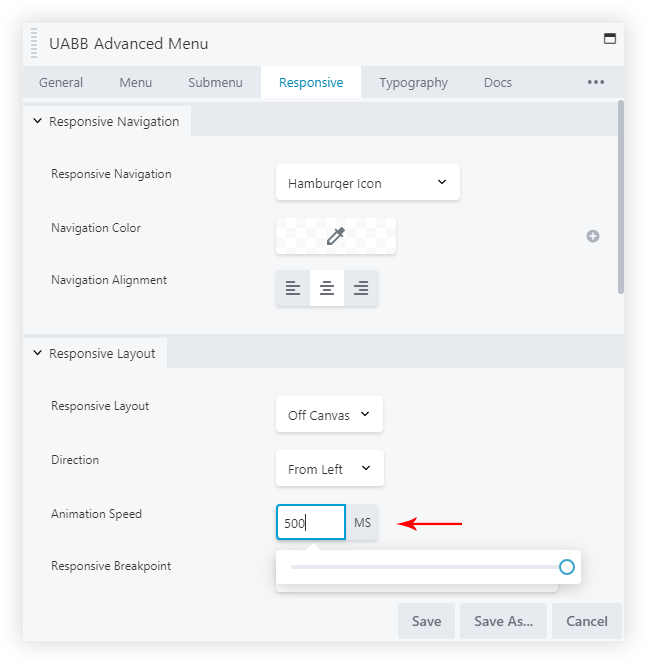The image displays the UABB Advanced Menu interface on a web page. The menu features several sections including General, Menu, Submenu, Responsive, Typography, and Documentation.

The currently selected section is "Responsive," highlighted with blue text against a white background, while other tabs are grayed out. Within the Responsive tab, there are several options:

- **Responsive Navigation:** This includes settings for a Green Dot, Responsive Navigation, a Hamburger Icon for dropdown menus, and Navigation Color, which can be adjusted using a rectangular color picker or a little pipette tool.
- **Navigation Alignment:** Options to align the navigation to the Left, Center, or Right.
- **Responsive Layout:** Choices include Off-Canvas layout and Typography settings.
- **Direction and Animation Speed:** Settings to control the direction from which the menu appears (Left) and the animation speed, set at 500 milliseconds (ms) with a right-pointing arrow indicating the unit.
- **Responsive Breakpoint:** A section with a large white bar inline for input.

At the bottom, there are buttons for Save, Save As, and Cancel. The overall page background is mostly gray with various text styles making up the interface. At the very top, there are several dash marks, suggesting a navigation breadcrumb or indicator.